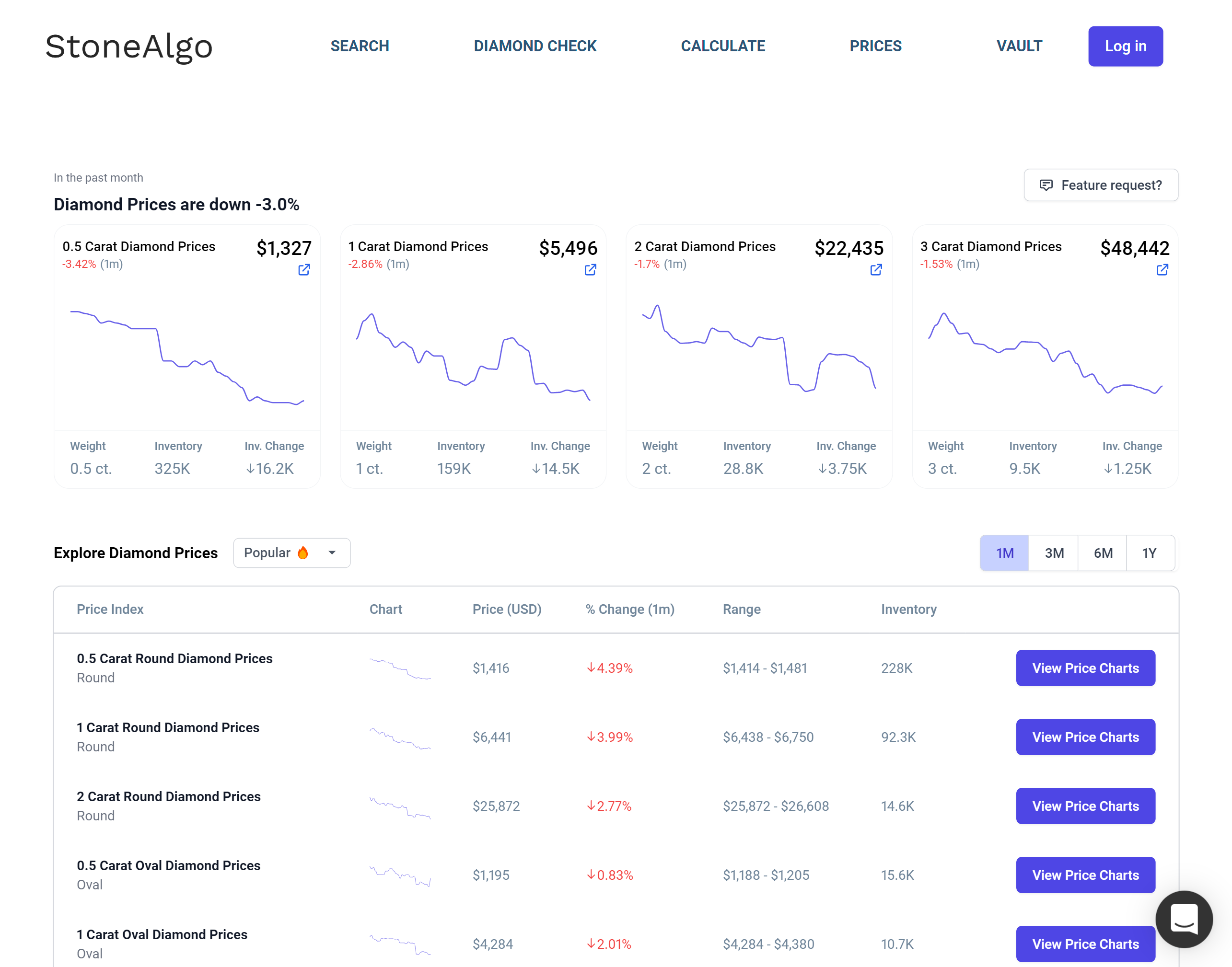The image showcases a webpage from StoneAlgo, a platform likely dedicated to analyzing and providing data on precious stones and diamonds. The central focus is on the recent trends in diamond prices, which have decreased by 3% over the past month. Various types of diamonds, differentiated by weight such as half a carat, one carat, two carats, and three carats, are all represented with individual graphs, indicating the declining trend in their prices over the specified time. Each graph visually portrays the consistent downward movement, although the half-carat diamonds show a slightly less volatile decrease.

Below these graphical representations, there is a detailed listing that includes current prices, the percentage change over the month, price ranges, and inventory figures. There are also buttons labeled "View Price Charts" for more in-depth analysis. At the top of the page, near the StoneAlgo logo, are navigation links for features such as search, diamond check, and price calculation, implying the site's specialization in diamond or precious gemstone market analysis. Additionally, users have the option to adjust the displayed time frames between three months, six months, or a year for broader historical data.